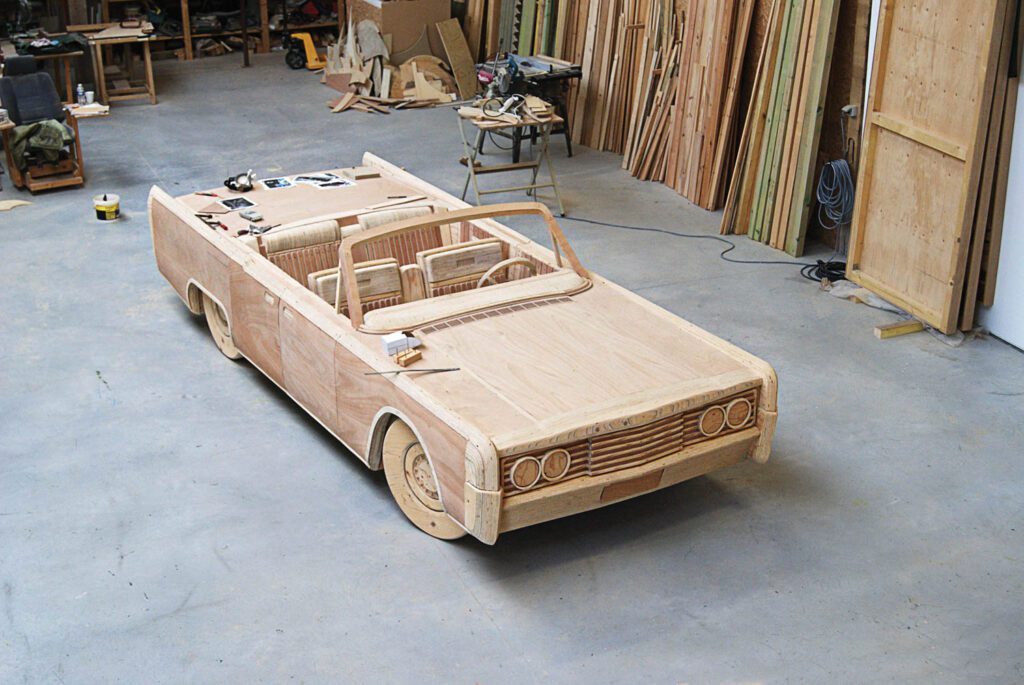The image features a detailed, life-size wooden model of a convertible car, situated in a spacious workshop or garage. The car, entirely made of wood—including its flat-topped body, wheels, and seats—faces slightly away from the camera, showcasing its side and front. Positioned on a concrete floor, the model is adorned with various items on its hood and trunk, such as photographs, plans, and possibly tools used during its construction. The background reveals an array of woodworking equipment: benches, tools, and numerous slabs of wood in different colors stacked against the walls, hinting at the craftsmanship and materials involved in the car's creation. The scene also includes a chair and additional scraps of wood, emphasizing the ongoing nature of the project.